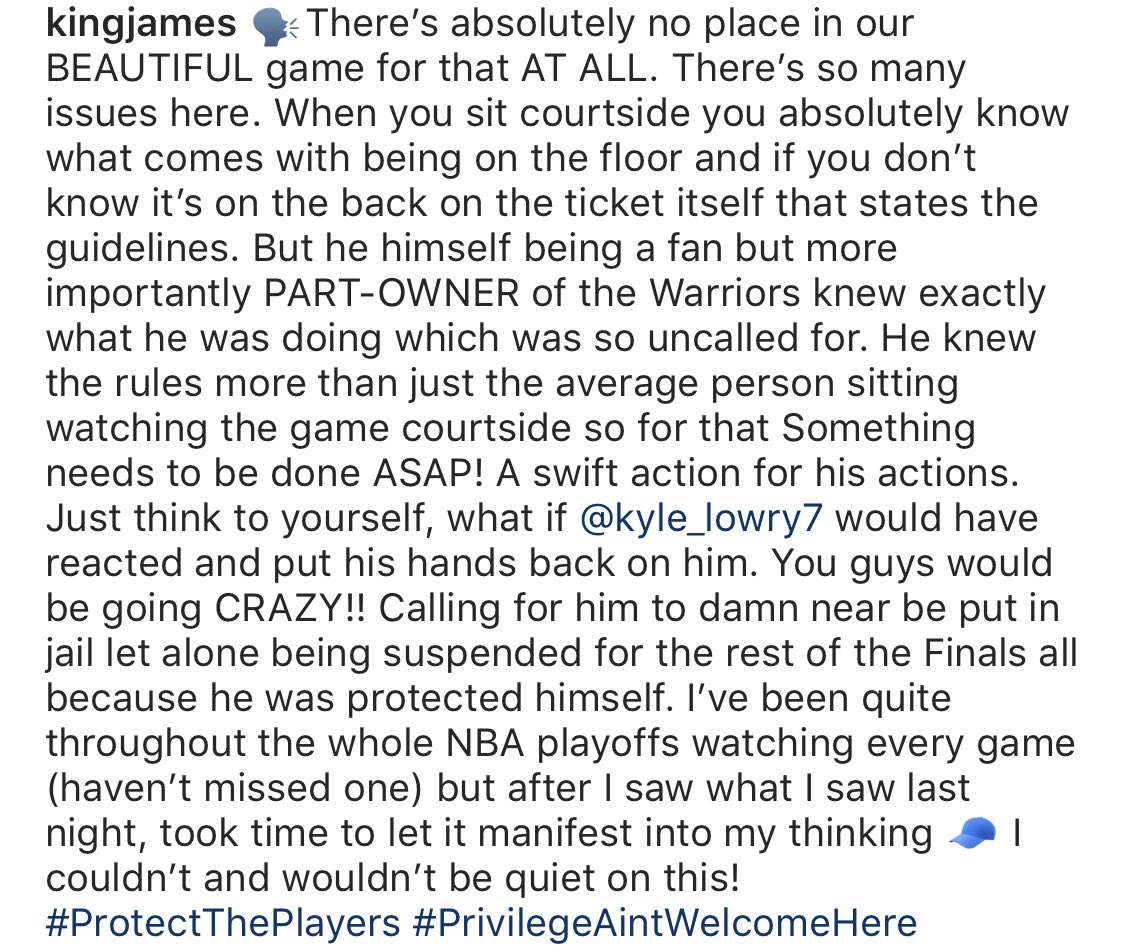The image captures a social media comment highlighting a stance on fan behavior during an NBA game. In the top left corner of the comment, "King James" is displayed prominently in bold black text, accompanied by an icon of a person speaking. The comment reads: "There is absolutely no place in our beautiful game for that at all. So many issues here: when you sit courtside, you absolutely know what comes with being on the floor. If you don't know, it's on the back of the ticket itself that states the guidelines. But he, being a fan, and more importantly, part owner of the Warriors, knew exactly what he was doing, which was so uncalled for. He knew the rules more than just the average person sitting courtside, so something needs to be done ASAP. A swift action for his actions. Just think to yourself, what if Kyle Lowry had reacted and put his hand back on him? You guys would be going crazy, calling for him to be damn near put in jail, let alone being suspended for the rest of the finals, all because he was protecting himself. I've been quiet throughout the entire NBA playoffs, watching every game."

The comprehensive comment delves into the expectations and responsibilities of courtside attendees, spotlighting the breach of conduct by a well-informed individual, and calls for immediate action, emphasizing the double standards in responses to player and fan interactions.